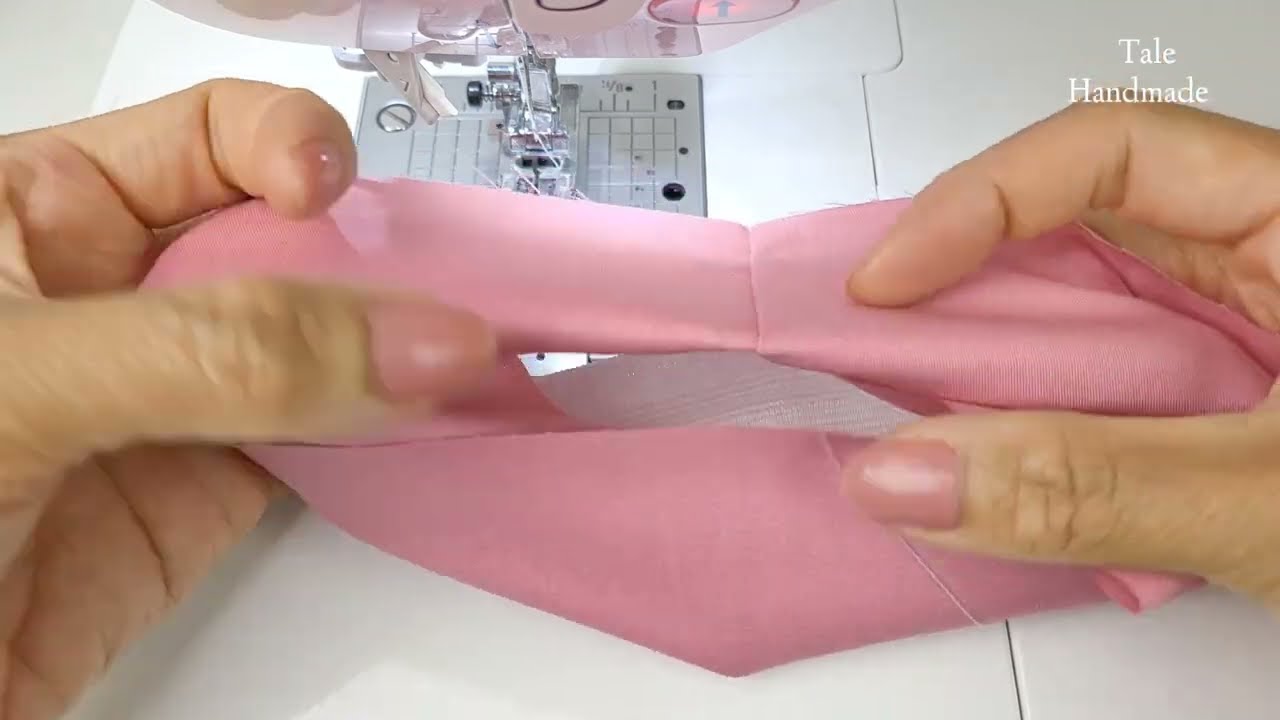The image is a detailed close-up of a sewing process, featuring two hands, possibly an older woman's due to slight wrinkles, meticulously working on a small piece of pink fabric. The hands, adorned with light pink fingernail polish, are positioned around the sewing machine's needle area, with the thumb and second finger on each side visible. The sewing machine itself is primarily white with a gray metal area around the needle mechanism, which includes a visible screw. In the top left corner, the text "TALE handmade" is displayed in white letters on two lines. This image likely originates from a sewing-related website or channel.